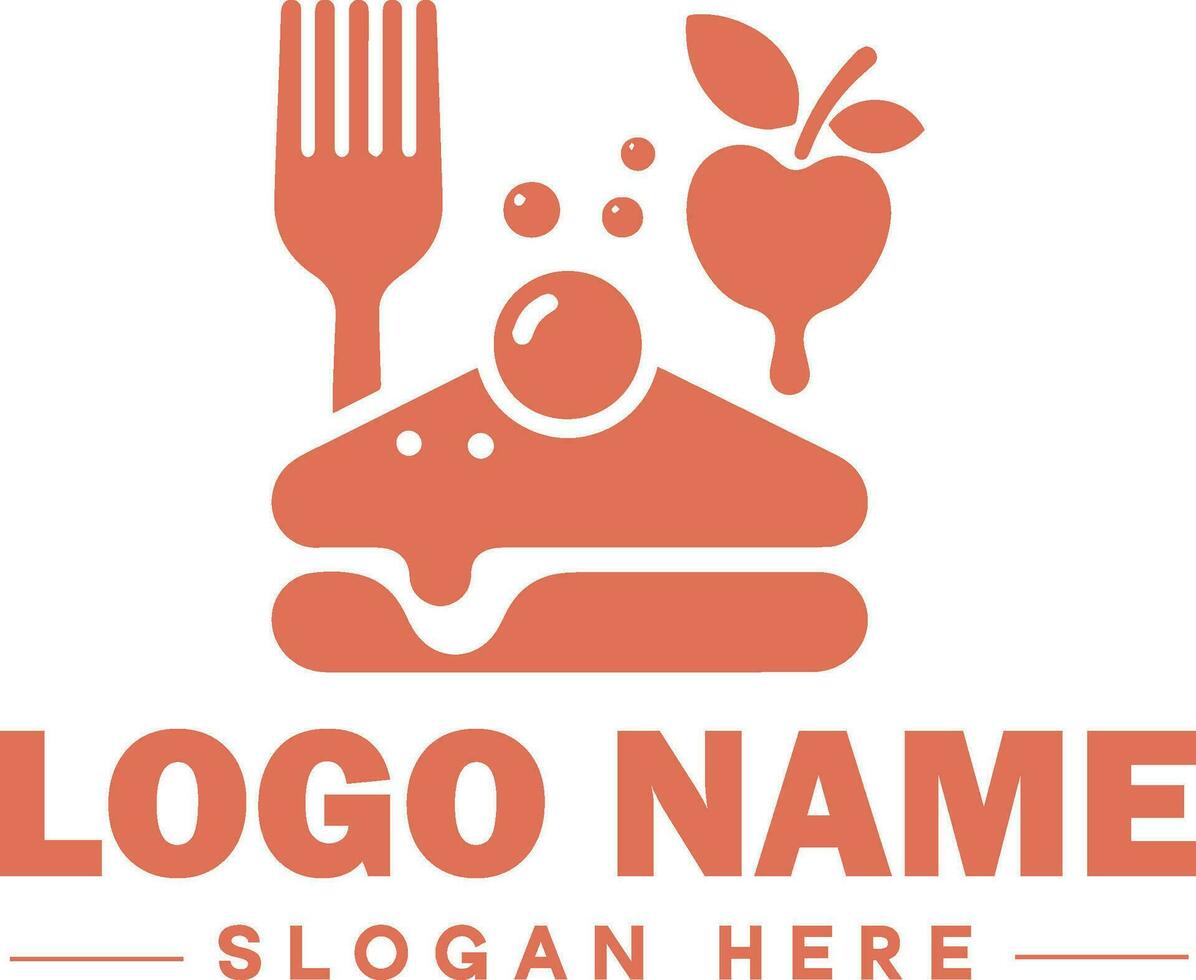This image depicts a detailed red-toned vector graphic on a white background, designed as a logo template possibly intended for a design or advertising company. Central to the graphic is a collection of monochromatic terracotta reddish-brown elements. 

On the upper left is a five-tined fork pointing upward. Next to the fork, slightly to the right, are three circles of varying sizes, each with a small white dot, suggestive of berries. Further right is a stylized apple drawing featuring a curved stem and two pointed oval leaves. Beneath these elements lies a diagonal representation of a half sandwich, marked by a triangular top layer with a garnishment circle, and a rectangular bottom layer, with a dripping detail that resembles cheese. 

Below these images, bold capitalized letters spell out "LOGO NAME." Directly beneath this, in smaller uppercase letters, is the placeholder text "SLOGAN HERE," flanked by horizontal lines on either side, all in the same terracotta hue. This visual template is likely a versatile stock photo or clip art, set up for custom company branding.